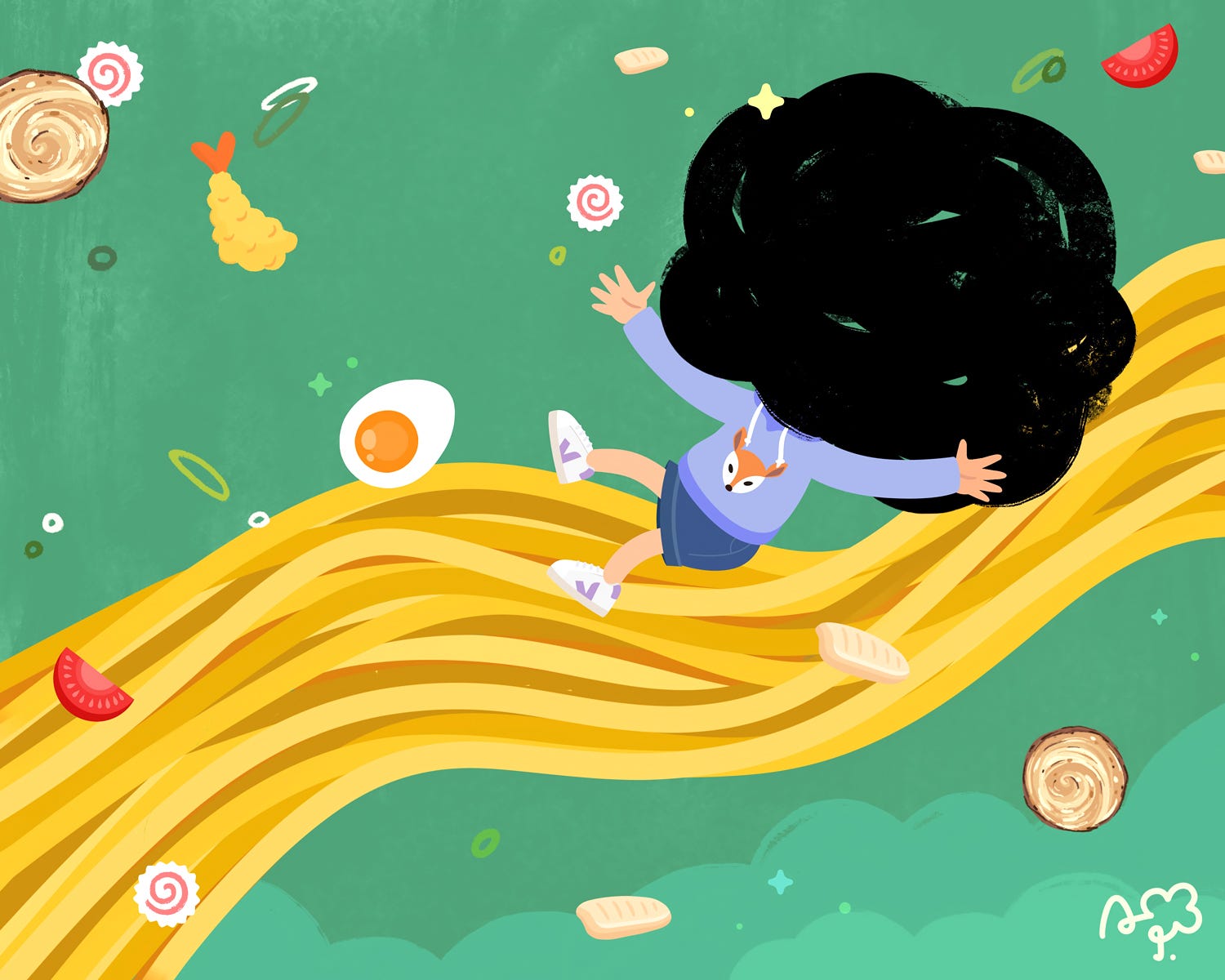This vibrant color illustration features a young girl sliding down a river of yellow ramen noodles that seem to flow in a wavy motion across the middle of the image. The background is predominantly green, interspersed with light green clouds towards the bottom. The girl, with her arms outstretched, wears a long-sleeved lavender hoodie adorned with an image of either a deer or a fox, a denim miniskirt, and white sneakers embellished with a purple 'V' pattern. Her legs are bare, and her head is obscured by a dense black cloud, creating an uncanny visual effect.

Surrounding the girl are floating ingredients commonly found in ramen, presenting a surreal scene: tomato wedges, fried shrimp, pieces of Naruto fish cake with red swirls, sliced hard-boiled eggs, green scallions, and an unidentifiable brown swirly circle. At the bottom of the image, the artist's stylized signature adds a final touch, though it's not legible. This unique artwork blends whimsical elements with a dash of mystery, making it a visually engaging piece.